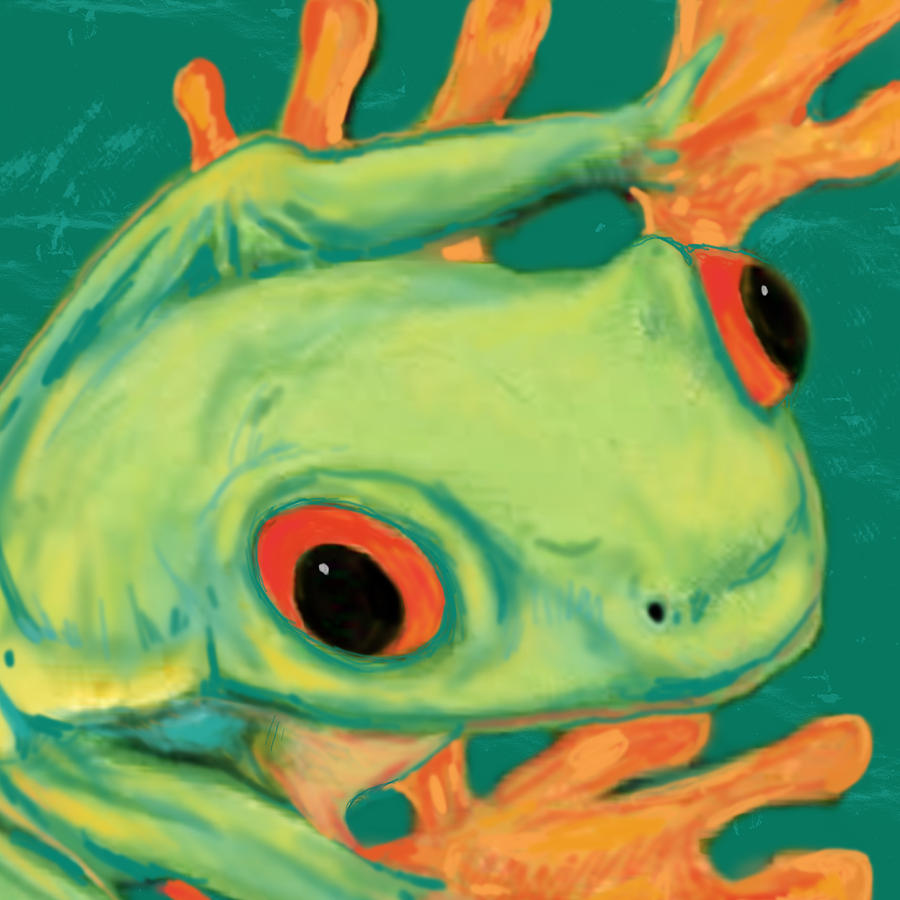The image depicts a pixel art rendering of a tropical frog prominently displayed in the foreground, occupying most of the frame. The frog's body is light green with darker green shadows that add depth to its appearance. Its eyes are bright red with large black pupils, which give it a bulging, attentive look. One visible nostril and a long, thin mouth are clearly detailed along the bottom of its head. The frog's feet are a striking bright orange, standing out vividly against green hues. The background, mainly a dark green, frames the frog with hints of aqua and teal highlights, accentuating the tropical setting. The frog, with its captivating red eyes and vibrant colors, appears to be staring directly at the viewer, creating an engaging and slightly mischievous presence.